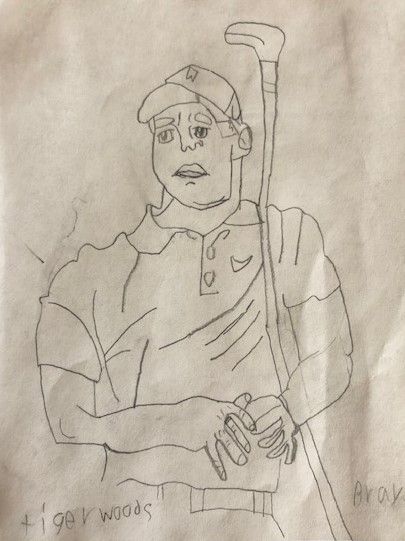This pencil drawing of Tiger Woods, created by Bray, features the golf legend standing and looking slightly to the left of the viewer. The artwork, done entirely in pencil, showcases Tiger wearing a hat and a golf shirt with two buttons, complemented by a belt. The shirt is detailed with plenty of texture, appearing bunched up and folded over. Woods holds a golf club, with the head of the club near his own head and the handle extending downwards, with his hands positioned together in front of his body. Notably, the proportions of the arms and hands are slightly off, particularly the fingers which appear somewhat distorted. Additionally, a ring is visible on his right hand. The drawing captures Tiger from the waist up and, while clearly an amateur piece, demonstrates earnest effort and potential for improvement.